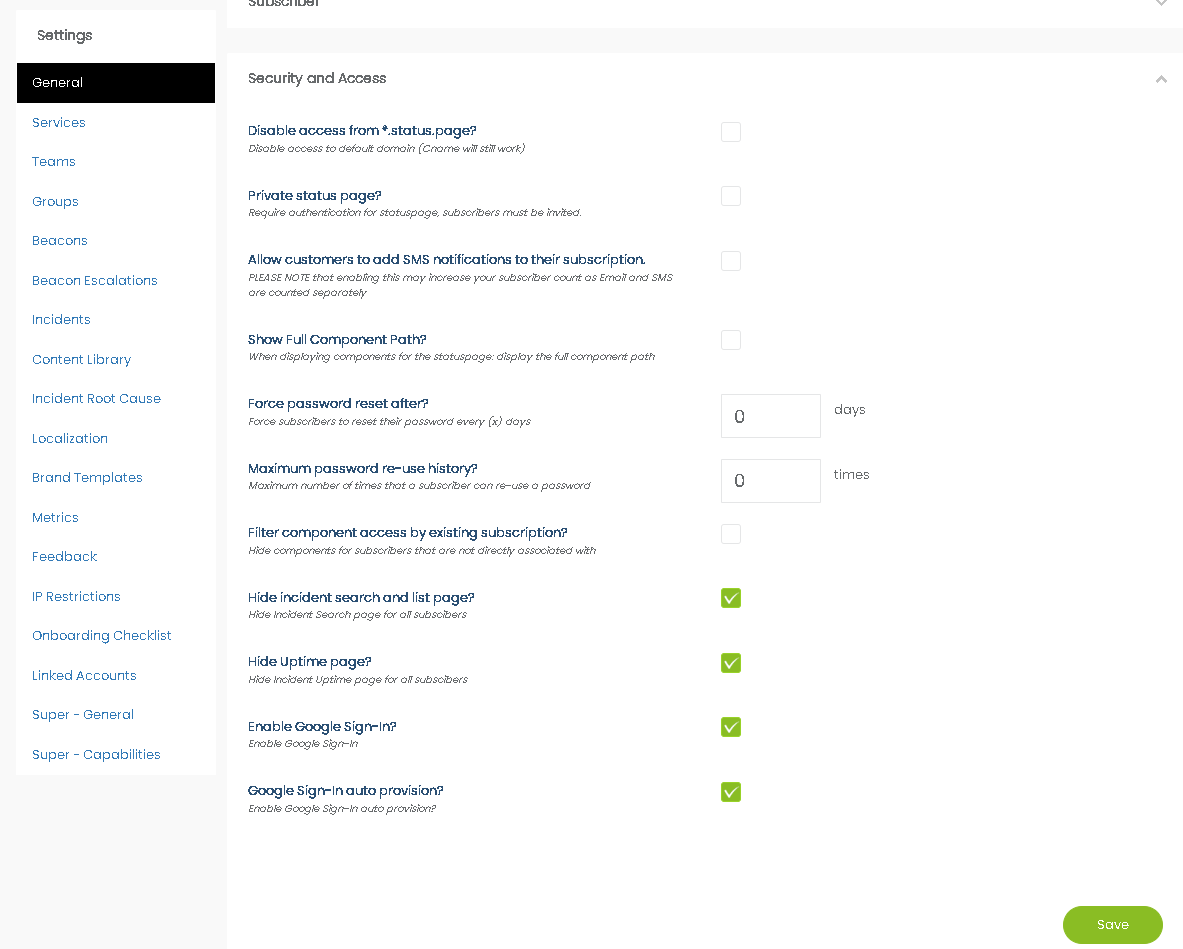This is a highly detailed screenshot of a settings page, showcasing a clean, white interface. On the left side of the screen, there is a vertical sidebar with a header labeled "Settings" in bold black text against a white background. Directly below the header, the option "General" is prominently highlighted with a black background and white text, indicating the currently selected section, while the rest of the menu items are in blue text. The sidebar menu includes several links: Services, Teams, Groups, Beacons, Beacon Escalations, Incidents, Content Library, Incident Root Cause, Localization, Brand Templates, Metrics, Feedback, IP Restrictions, Onboarding Checklist, Linked Accounts, Super General, and Super Capabilities.

The main section of the page, situated to the right of the sidebar, focuses on security and access settings. It features an option titled "Disable Access from Status Page" with an adjacent checkbox. Below it, there's another option labeled "Private Status Page," also with a checkbox. Each listed option comes with checkboxes, which are either blank or marked with a green checkmark, indicating whether the respective feature is enabled or not. The overall design is clean and organized, with a clear distinction between different sections and settings for ease of navigation.